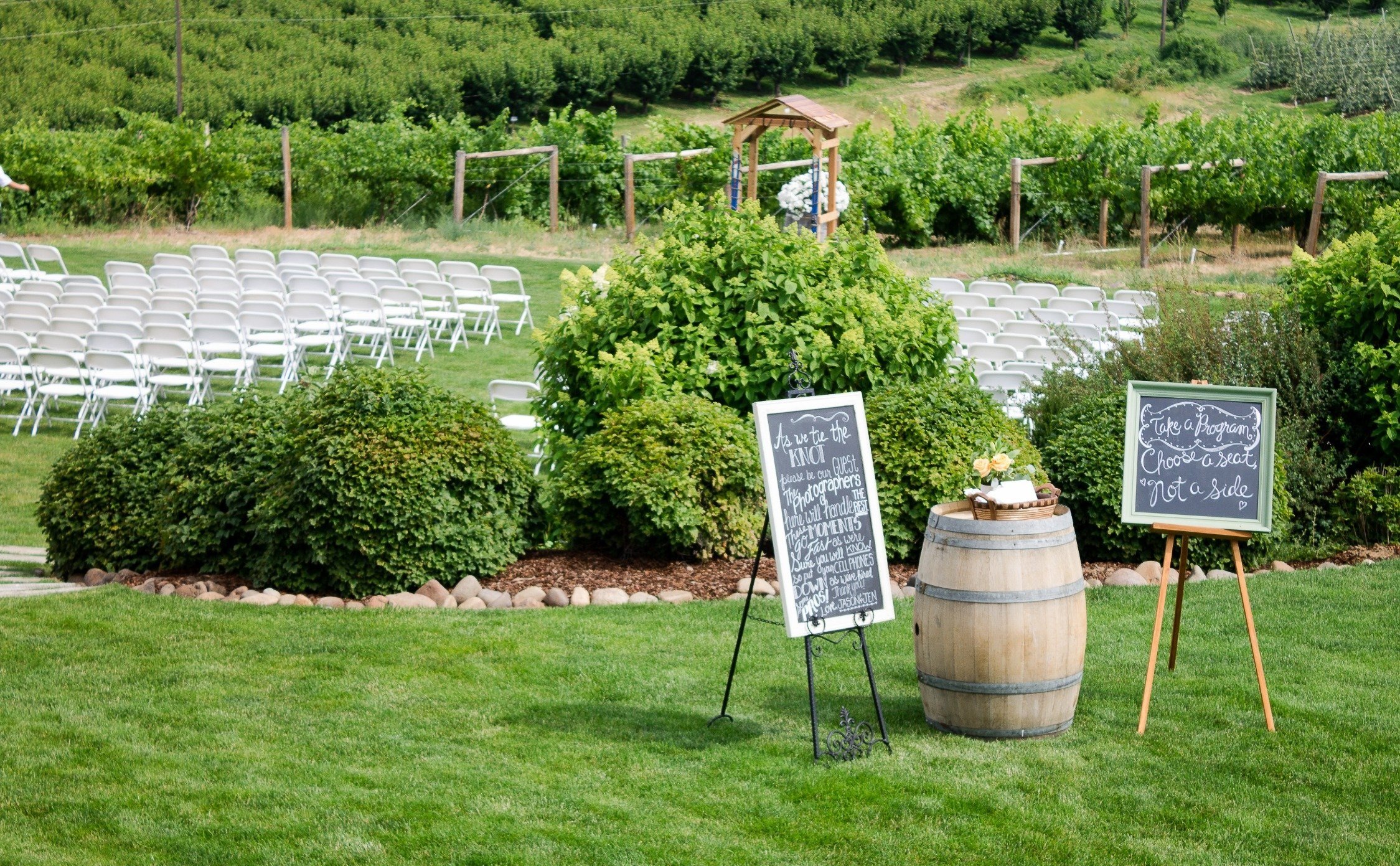The photograph depicts a picturesque outdoor wedding venue set within a verdant wine vineyard. In the foreground, there are approximately 12 rows of white folding aluminum chairs, arranged 10 across, situated on a lush green lawn that slopes gently downward. To the left, a black wrought iron easel displays a white-bordered wooden sign with partially legible chalk writing that reads, "As we tie the knot." On the right-hand side, a brown wooden easel holds a green-framed chalkboard sign that clearly instructs guests, "Take a program, choose a seat, not a side."

At the right corner of the image, a white wine cask barrel decorated with a small basket contains white cards, likely wedding programs. Centrally positioned in the background, a quaint brown gazebo adorned with white flowers stands ready to host the ceremony. The gazebo is surrounded by neatly trimmed green shrubbery and scenic landscaping, with rows of vineyard plants visible further up the hill, reinforcing the winery setting. A road runs parallel to the vineyard, framing the charming and well-maintained venue.